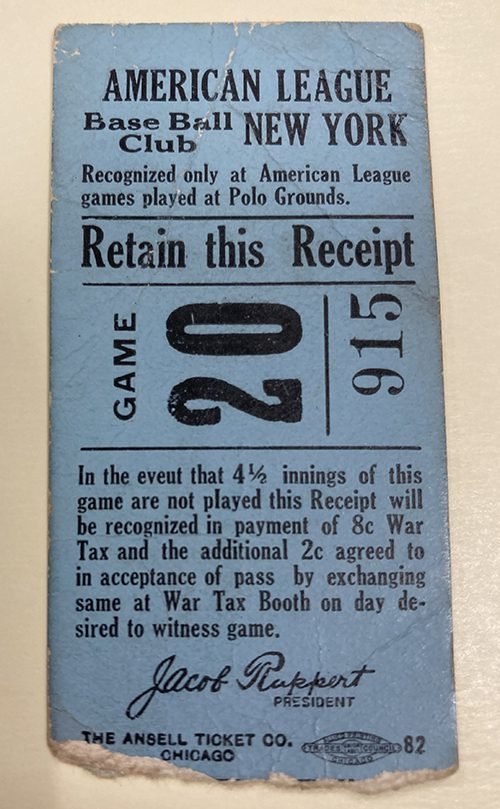This photograph showcases a vintage sky blue ticket stub from an American League Baseball Club game in New York, specifically for Game 20 held at the Polo Grounds. The aged ticket, signed by Jacob Ruppert, the club's president, includes seat number 915 and features distinctive text detailing that it is only recognized for American League games at this venue. A notable detail indicates that if fewer than four and a half innings were played, this receipt could be exchanged, recognizing an eight-cent war tax and an additional two cents at a designated war tax booth. The stub also shows wear and tear, with parts missing at the bottom and some text revealing white under the blue surface. The ticket is lying on a bone-colored backdrop, highlighting its historical significance and well-worn condition from frequent handling. The name "Andal Ticket Company, Chicago" is printed on it, potentially indicating the origin of its manufacture.